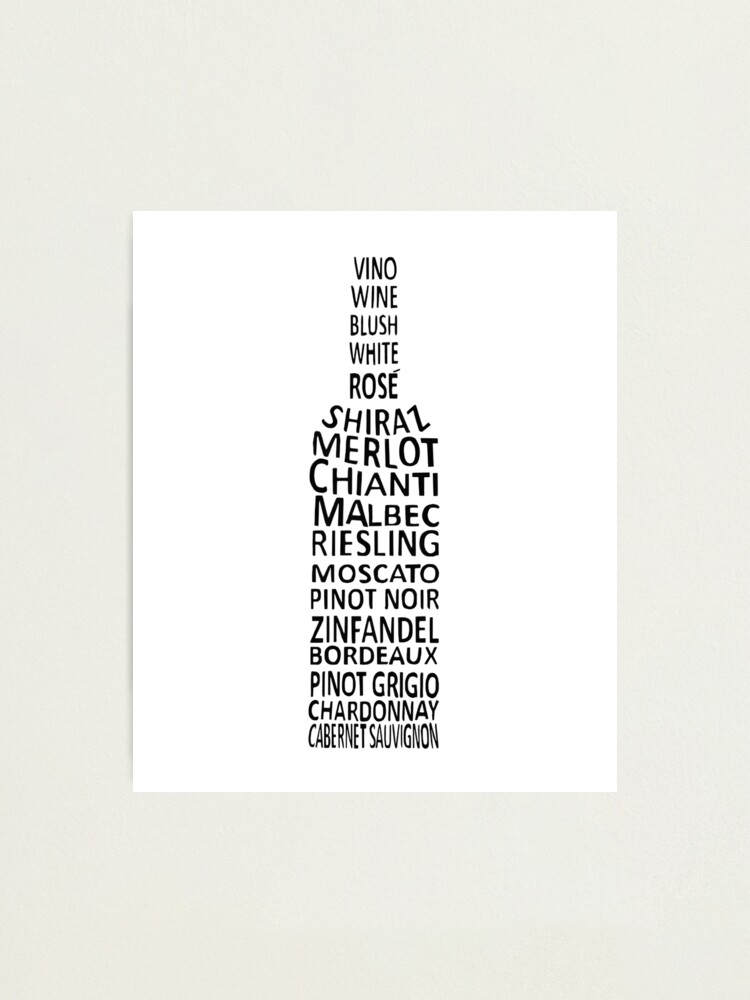This image is a promotional graphic cleverly designed using black text on a white background, featuring various words associated with wine, arranged to form the cylindrical shape of a wine bottle. Dominantly centered on what appears to be a white canvas against a light gray background with a subtle drop shadow on the left, the layout draws immediate attention. The text starts from the top with "vino," followed by "wine," "blush," "white," "rosé," "Shiraz," "Merlot," "Chianti," "Malbec," "Riesling," "Moscato," "Pinot Noir," "Zinfandel," "Bordeaux," "Pinot Grigio," "Chardonnay," and ending with "Cabernet Sauvignon" at the base. The font size varies, with smaller text at the neck of the bottle and larger text at the body, enhancing the visual representation of a wine bottle. This creative composition highlights the diverse wine varieties and is strikingly hung on the wall, making the bottle the central focus while maintaining a clean and minimalist aesthetic with ample white space.